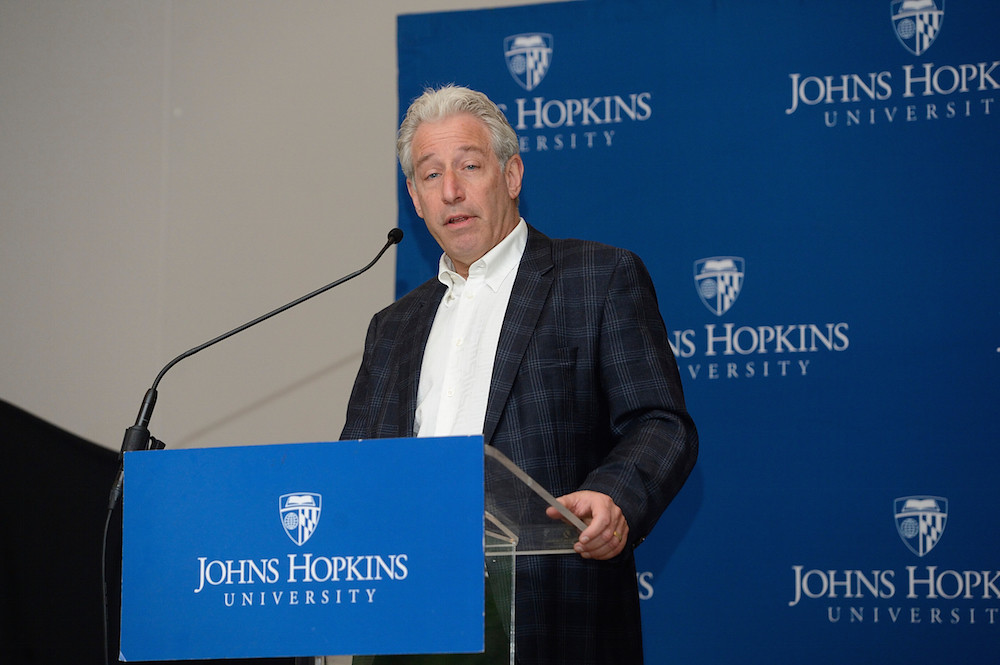This photograph captures an older man, aged between 50 and 65, speaking at a podium at Johns Hopkins University. The man, who is white with gray hair and blue eyes, is smartly dressed in a dark suit and a white button-down dress shirt. He stands behind a transparent podium adorned with a blue sign bearing the Johns Hopkins University logo. The microphone is attached to the podium and pointed towards his mouth. The backdrop behind him is covered with repeated logos and the words "Johns Hopkins University." To his left, part of the wall is visible; it is brown at the top and black at the bottom. The man is looking to the left as he addresses his audience.